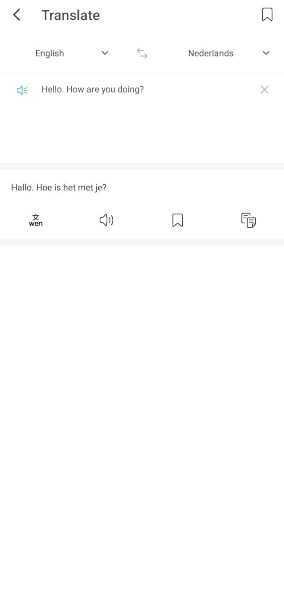The web page features a minimalist design on a white background. Central to the interface is a series of translation tools and informational elements. 

At the top left, a black left-pointing arrow is labeled "Translate" in black text. On the far right, a black bookmark icon is present. Below this, there is a white rectangular field labeled "English," accompanied by a black drop-down arrow for language selection. Adjacent to it, another gray drop-down arrow is next to the word "Netherlands" (likely intended to be "Dutch"), indicating the target language selection.

The main content area showcases a white text box with teal speaker icon emitting teal lines to signify sound. Inside the box, the text reads in black: "Hello. How are you doing?" A black or gray 'X' icon is situated at the top right corner of this box for dismissal.

Below, additional translation results appear. In bold black text, it says "H-A-L-L-O," followed by "H-O-E" and "het met J-E?" This translates the English phrase into Dutch. A description beneath this indicates the translation process between English and Dutch.

A series of icons follow: a star labeled "W-E-N" in bold black text, a teal speaker icon, a blue clipboard icon, and two black paper icons with a gray band underneath.

The image is cropped, leaving out any additional context from the edges.